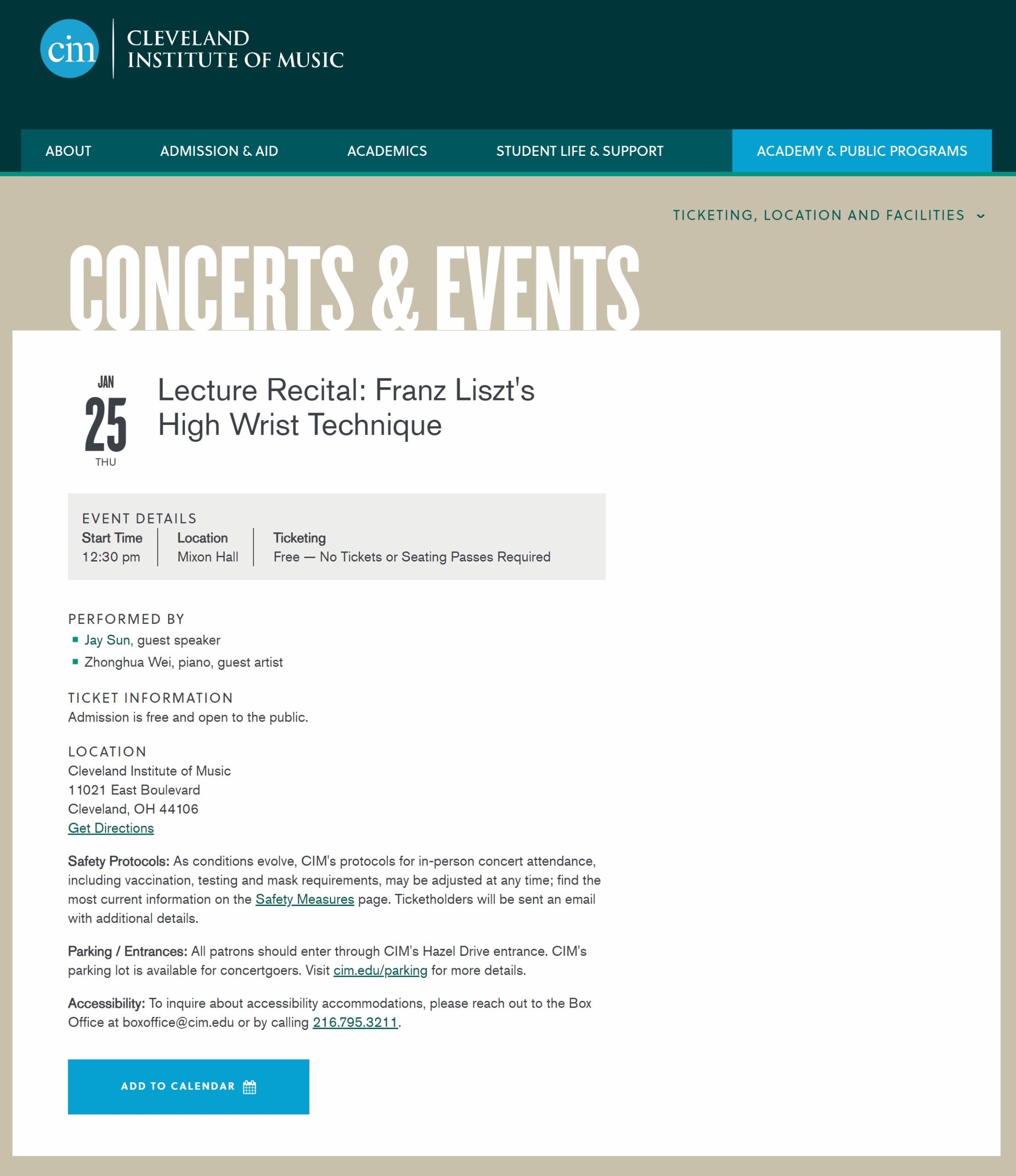Screenshot of the Cleveland Institute of Music website. Below the institution’s logo, a green menu section is visible with categories labeled: About, Admission and Aid, Academics, Student Life and Support, and Academy and Public Programs. The page is titled "Concerts and Events." There is a listing for an event on Thursday, January 25th, featuring a Lecture Recital on "Franz Lentz: High Wrist Techniques." The event begins at 12:30 PM and will be held at Mixon Hall. Admission is free and no tickets or seating passes are required. The lecture recital will be delivered by guest speaker and pianist Jay Sun.